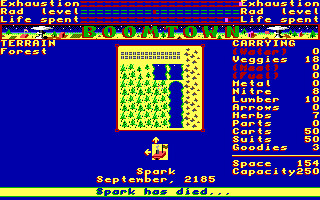This image is a nostalgic screenshot of a vintage video game, possibly from the 1980s, set in a predominantly blue background. The game title "Boomtown" is prominently displayed in green capital letters at the very top center of the screen. The upper-left and upper-right corners both feature the words "Exhaustion," "Rad Level," and "Life Spent."

Just beneath the title, there's a detailed yellow grid-like square with a red border, containing simplistic green representations of trees and blue squiggly lines that likely depict water. This square encapsulates the terrain labeled "Forest."

To the right side of the image, there is a vertical list under the heading "Carrying," enumerating items and their quantities: "Water (0)," "Veggies (18)," "Meat (0)," "Fuel (0)," "Metal (0)," "Nature (8)," "Lumber (10)," "Arrows (0)," "Herbs (7)," "Parts (0)," "Carts (50)," "Suits (50)," and "Goodies (3)." Beneath this list, it reads "Space 154 Capacity 250."

At the very bottom, it states "Spark, September 2185," in yellow text with a smaller green yellow-dyed spark icon. It adds a somber note with "Spark has died..." suggesting the end of a game session.